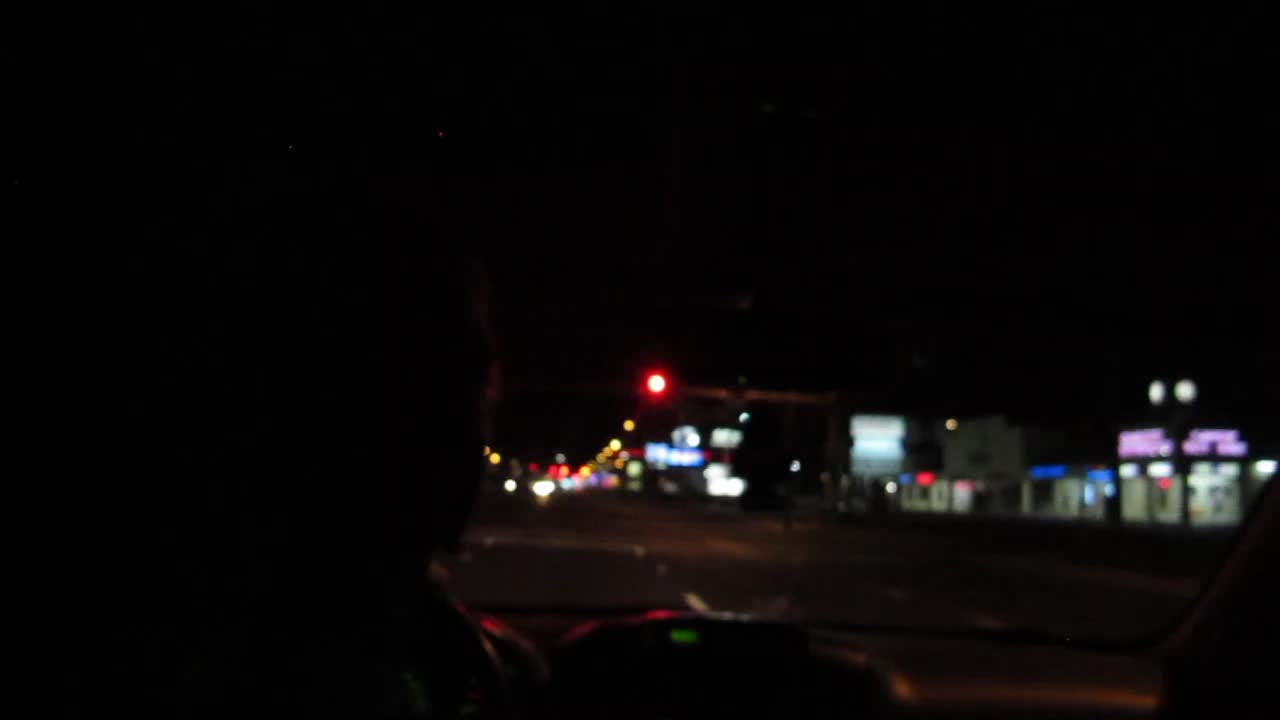A nighttime scene captured through the windshield of a vehicle, likely from the back seat, revealing part of the driver with curly hair on the left. The driver's profile is partially illuminated, while the smooth, gray dashboard on the bottom right is subtly lit by ambient light. The car is traveling on a dimly lit road with sparse traffic; in the distance, blurry white headlights of oncoming cars are seen. An approaching red traffic light casts a faint glow on the surroundings. To the right, a row of buildings resembling a strip outlet is adorned with neon signs and purple lights, adding a splash of color to the predominantly dark scene. Further ahead, scattered yellow lights from street lamps or building illuminations punctuate the blackness, creating a moody and serene atmosphere.